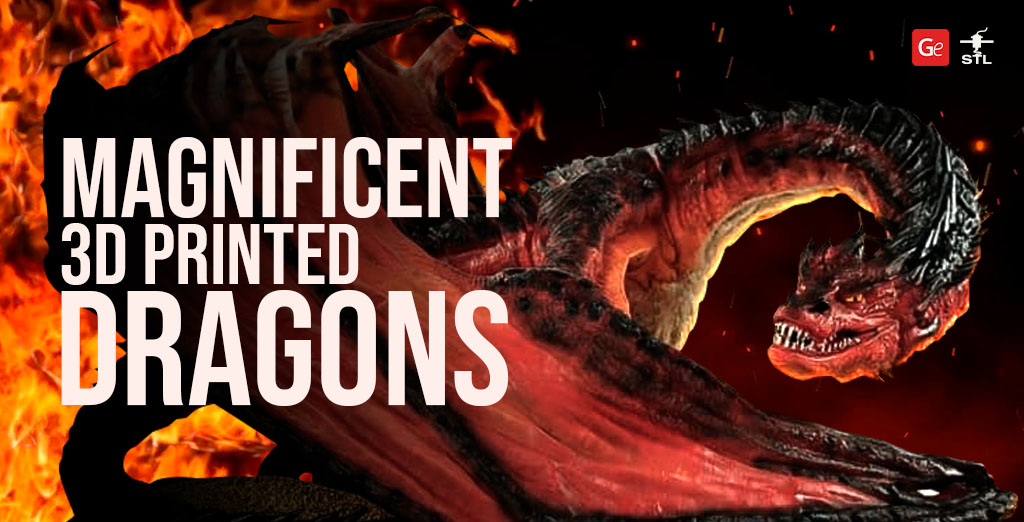The advertisement banner features a dynamic and captivating design, set against a dark black and reddish background with vivid flames. Central to the image is an intricately detailed 3D-printed dragon, painted in deep, dark red hues. The dragon's black spines add to its menacing appearance, while its large, red wings extend behind the prominently displayed text. The dragon is posed realistically, with its body side-facing and its head curving around to meet the viewer's gaze. Its belly contrasts in a light yellow color, starting from under its neck.

The text overlay is composed of bold, all-capital, sans-serif letters. At the top, the word "MAGNIFICENT" stands out in white, followed by "3D PRINTED" in a smaller font, and then "DRAGONS" in a larger size, emphasizing the grandeur of the dragon.

In the top-right corner, there is a small red square featuring the letters "GE" next to an icon, indicative of a logo, with the letters "STL" written below it in white. The left side of the banner showcases a wall of intense flames, while the right side transitions from black to red, scattered with sparks and specks of flames, adding a dynamic and fiery ambiance to the scene.